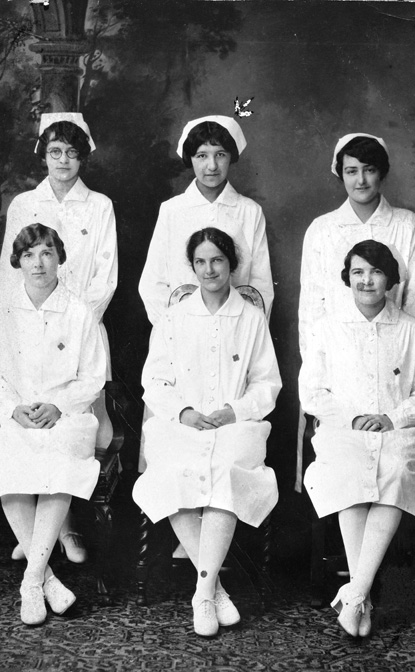This black and white photograph, likely taken 30-40 years ago, features six nurses, possibly commemorating their graduation. The image is meticulously posed, with three nurses seated in front and three nurses standing directly behind them. The seated nurses, dressed in pristine white uniforms complete with white stockings and shoes, have their hands gracefully crossed in their laps and their legs elegantly crossed as well. From left to right, the seated nurses exhibit diverse hairstyles: the nurse on the left has wavy, short hair; the nurse in the center has her hair pulled back; and the nurse on the right has short hair. Each seated nurse is mirrored by a standing nurse behind her, all adorned in matching white uniforms and traditional white nurses' caps. Notably, the nurse standing on the left wears glasses. The background reveals a wall adorned with varied textures, resembling a large painting. On the left side of the wall, there's a detailed image of a column flanked by trees and foliage. The foreground showcases an ornate carpet beneath the nurses' feet, contributing to the refined and formal atmosphere of the photograph.